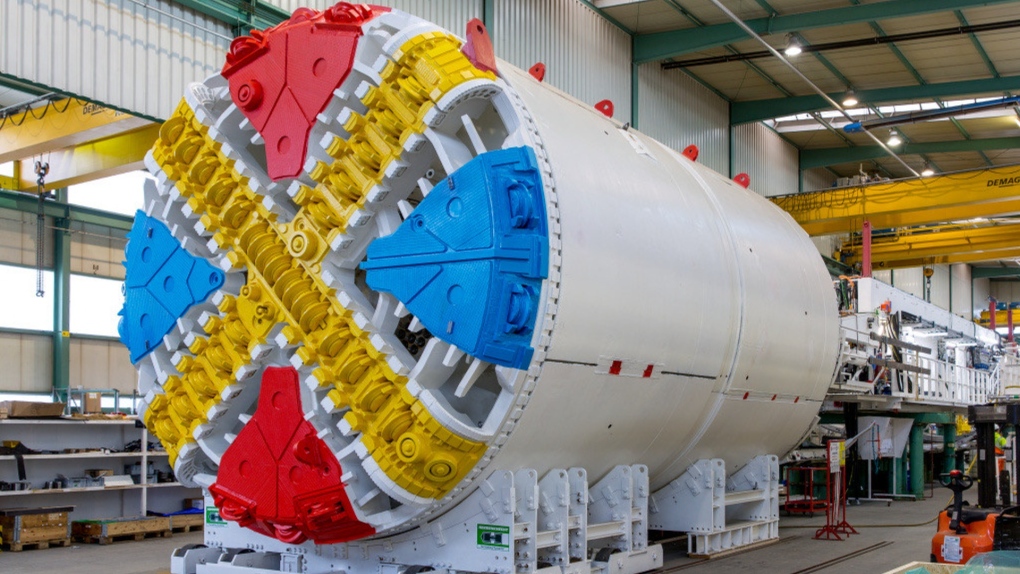The image captures a large, horizontally positioned white cylinder placed inside a spacious warehouse. The cylinder appears to be a sophisticated mechanical or scientific device. On the side of the cylinder, there is a prominent yellowish X formed by various intricate components. Complementing this feature are two blue triangular sections on the left and right sides and two red triangular sections on the top and bottom sides of the X. The cylinder is supported by sturdy white beams.

The warehouse itself is characterized by green ceiling supports and white, ribbed walls. The ceiling is also white and features black poles with attached lights. Yellow beams are visible around the space, adding structural detail. A white structure can be seen in the background on the right side of the image. Additionally, there are windows on the right side of the building and a collection of tools neatly arranged on shelves at the bottom left side of the scene.